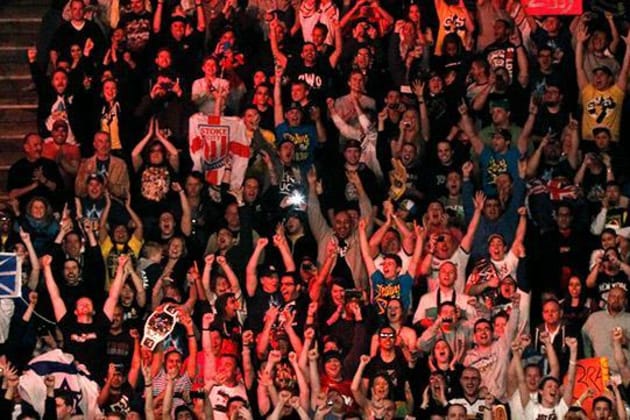This color photograph captures a lively group of predominantly young male spectators packed into the stands of a sports arena or stadium. The crowd's arms are enthusiastically raised high in the air, and their open mouths and animated expressions suggest they are cheering fervently, possibly reacting to a pivotal moment like a score or a band performance. The scene is filled with a mix of monochromatic black shirts and vibrant red and reddish shirts, indicative of the team's or band's colors. Multiple signs are visible throughout the audience, including a red sign partially cut off in the top right, an orange and yellow sign in the bottom right, and a distinct red and white sign towards the upper left middle. Additionally, a bright flash from a cell phone camera is prominently captured in the center of the image. The venue’s concrete steps are slightly visible on the left side, and one spectator is even holding up a wrestling belt, hinting at the possibility this could be a wrestling event. Overall, the atmosphere is electric with excitement, suggesting this could be a sports event, wrestling match, or high-energy concert, with the crowd possibly aware they are being filmed or photographed for a big screen, adding to their exuberance.